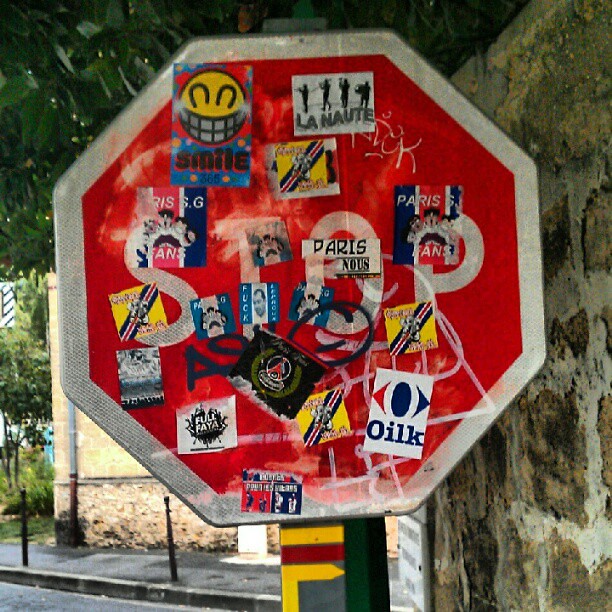This photograph captures a heavily weathered stop sign, almost entirely obscured by an assortment of stickers and graffiti, rendering its original red and white coloring nearly unrecognizable. The sign is plastered with various political and vulgar stickers, as well as advertisements, including one for a marching band. Among the stickers, several reference Paris, suggesting the sign's location in France, while others relate to soccer. A couple of stickers bear cheerful messages like "Smile," alongside some with foul language. The stop sign appears worn, with evidence that maintenance workers have repeatedly attempted to scrape off the stickers. In the background, an old-fashioned brick and stone wall is visible, complementing a likely church-like structure partially obscured by a lush array of trees and bushes. A tree branch hangs down close to the top of the stop sign, adding to the urban yet somewhat historic city ambiance. The scene also includes a sidewalk and part of a street, completing the intricate urban landscape.